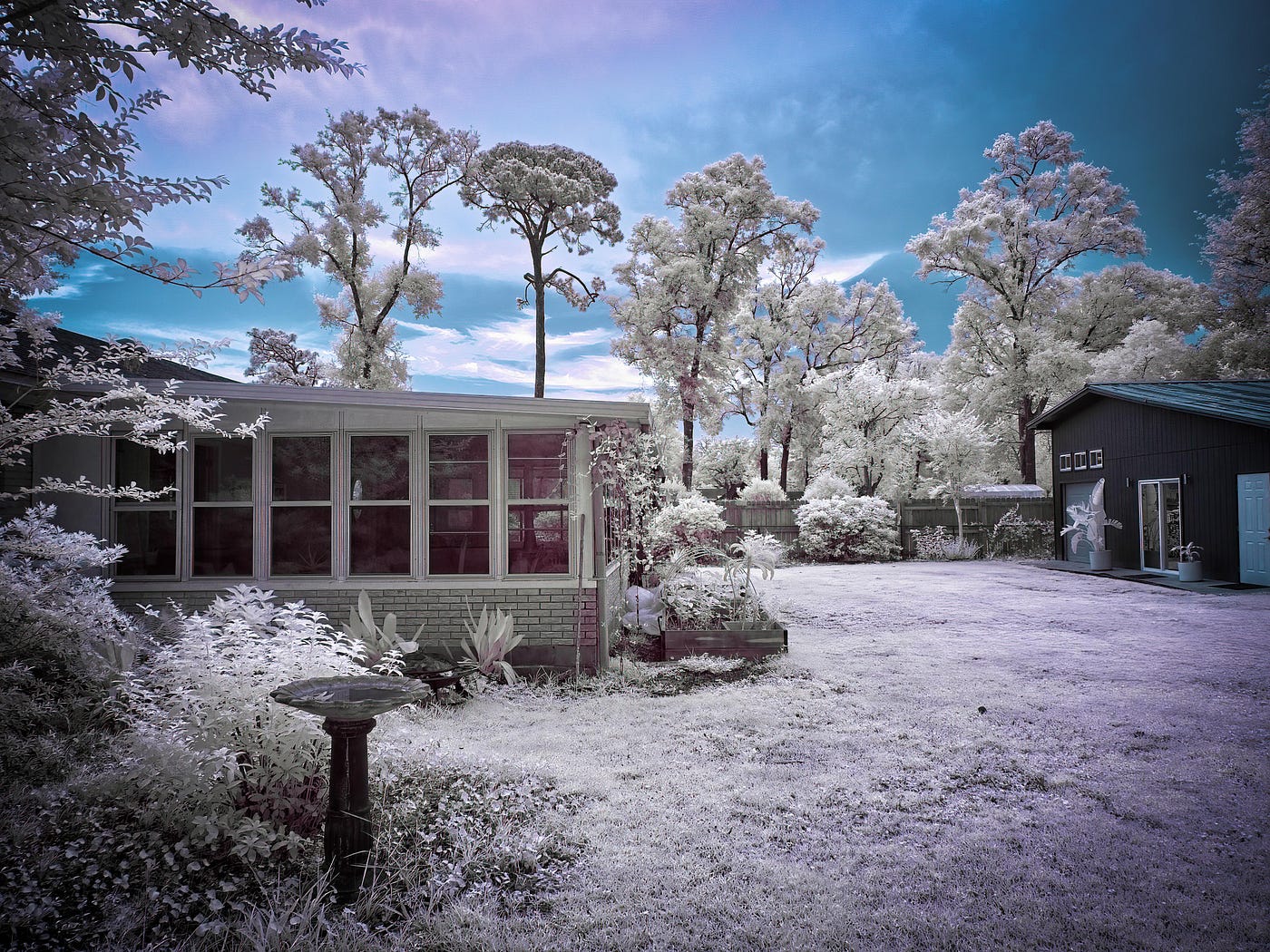The photograph features a surreal, slightly dreamy outdoor scene dominated by a brick, one-story house with numerous windows on the left side and a brown shed or secondary structure on the right. The grassy lawn in the foreground, oddly colored in a mix of grayish green and light purple, adds to the fantastical feel of the image. The vibrant steel blue sky with clouds enhances the unnatural atmosphere, visibly altered through photo editing. Trees in the background appear ghostly with white or very light green leaves, giving an impression of being coated in ice or snow. The yard, framed by a brown and white fence, displays additional bushes seemingly covered in icy coatings. This manipulated, artificial color palette creates a surreal and vivid scene that does not align with typical natural colors.